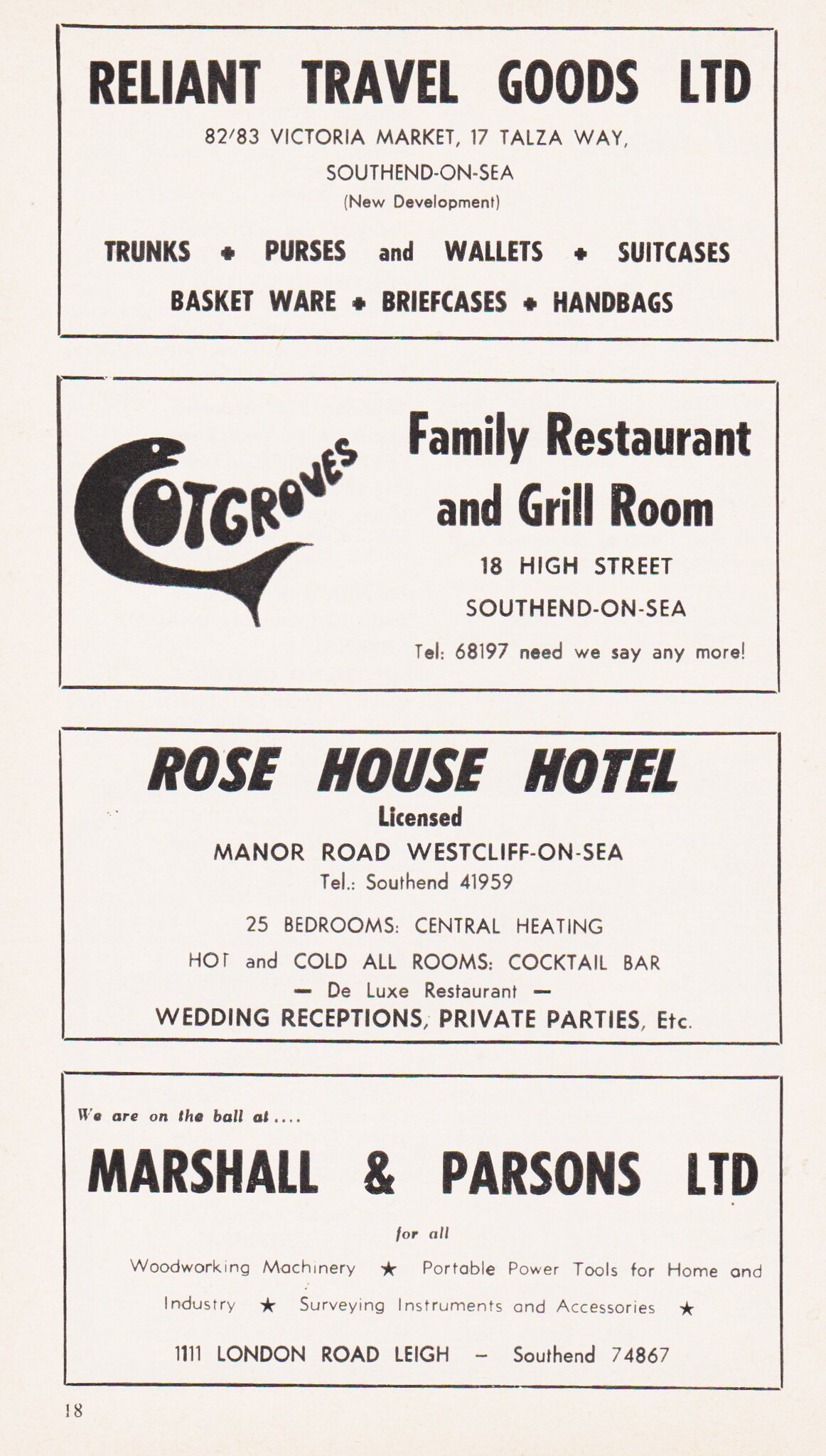This black-and-white photograph captures four vintage advertisements, likely from a local magazine or newspaper dating back 50 to 100 years. Each advertisement is neatly sectioned into a rectangle, prominently featuring the businesses in bold fonts and detailed descriptions.

At the top, the ad for Reliant Travel Goods, LTD is displayed. It lists their address at 82-83 Victoria Market, 17 Towsaway, Southernd-On-C, and details their wide range of travel goods including trunks, purses, wallets, suitcases, basketware, briefcases, and handbags.

Below that, there's an advertisement for Gott Groves, a Family Restaurant and Grill Room. Located at 18 High Street, Southernd-On-C, the ad includes their telephone number, 68197, and features the playful slogan "Need We Say Anymore?" The logo creatively incorporates a fish into the design of the letter "C".

Next is the ad for the Roadhouse Hotel, situated on Manor Road, Westcliff-On-C. The hotel boasts 25 bedrooms, central heating, and hot and cold water in all rooms. It also offers a cocktail bar, deluxe restaurant, and facilities for wedding receptions and private parties. Contact information is listed as Southernd-41959.

The final ad is for Marshall & Parsons LTD, located on London Road Lay, Southernd. They specialize in woodworking machinery and portable power tools for both home and industry, with their contact number being Southernd-74867. The ad highlights their expertise with the slogan "We Are On The Ball At Marshall & Parsons LTD".

Overall, these advertisements provide a nostalgic glimpse into the commercial life of Southernd, showcasing a diverse array of services and goods from travel essentials to dining, hospitality, and specialized tools.